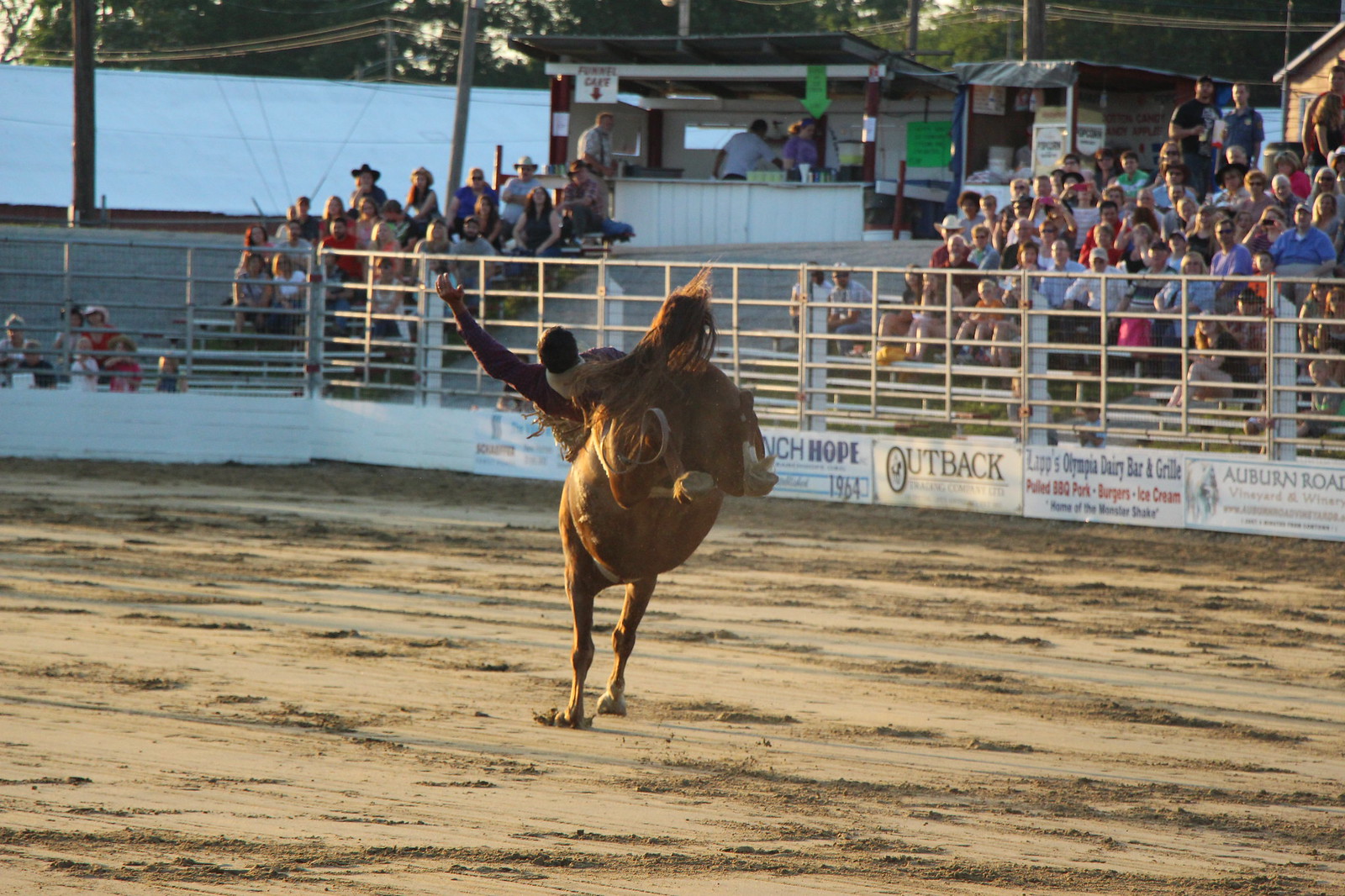The image captures a dynamic rodeo scene in an outdoor setting, centered on a bucking horse in a dirt arena. The horse, with its front hooves planted firmly on the ground and its back legs kicked high into the air, is attempting to throw off its rider. The rider, dressed in typical rodeo attire with black hair visible, has one arm outstretched and is precariously leaned back along the horse’s back, emphasizing the struggle to stay mounted. Surrounding the arena is a sturdy fence adorned with advertisements, including prominent ones for "Outback" and "Auburn Road." Beyond the fence, enthusiastic crowds are seated in bleachers that extend 10 to 15 rows high, attentively watching the thrilling event unfold. A concession stand is visible at the top of the stands, indicating it's a well-attended event. The background includes a few trees and poles, framing the arena on what appears to be a bright, sunny day. The overall composition suggests a professionally captured moment, with everything well-framed and clearly lit.